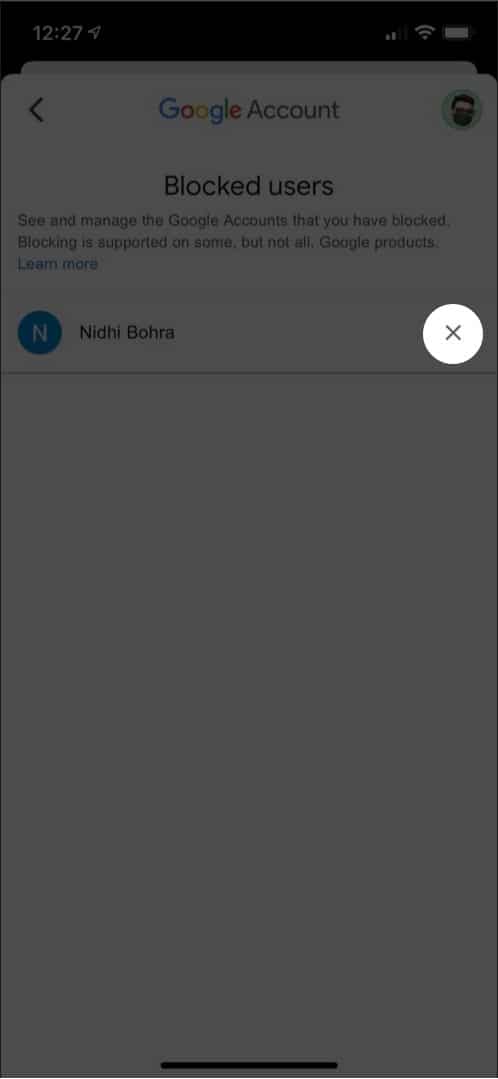The image depicts a smartphone screen displaying a "Google Account" settings page. At the very top, there's a black status bar showing the time (12:27 on the left), along with Wi-Fi signal strength and a fully charged battery symbol on the right. Below the status bar, the screen transitions to a predominantly white background.

At the top of this white section, the header reads "Google Account" on the left, with a circular icon on the right that features a faint gray outline resembling a person with a beard. Beneath this header is a section titled "Blocked Users," accompanied by a description that reads, "See and manage the Google Accounts that you have blocked. Blocking is important and supported on some, but not all, Google products." There is also a "Learn More" link below this description for additional information.

Following this, there is a listing displaying blocked individual(s) with a blue circle containing a white 'N' on the left, indicating a profile icon. The name "Nidhi Bhora" is written beside it, and on the far right, there is a white circular button with an 'X' symbol, likely for unblocking this user. The rest of the screen below this entry is blank.